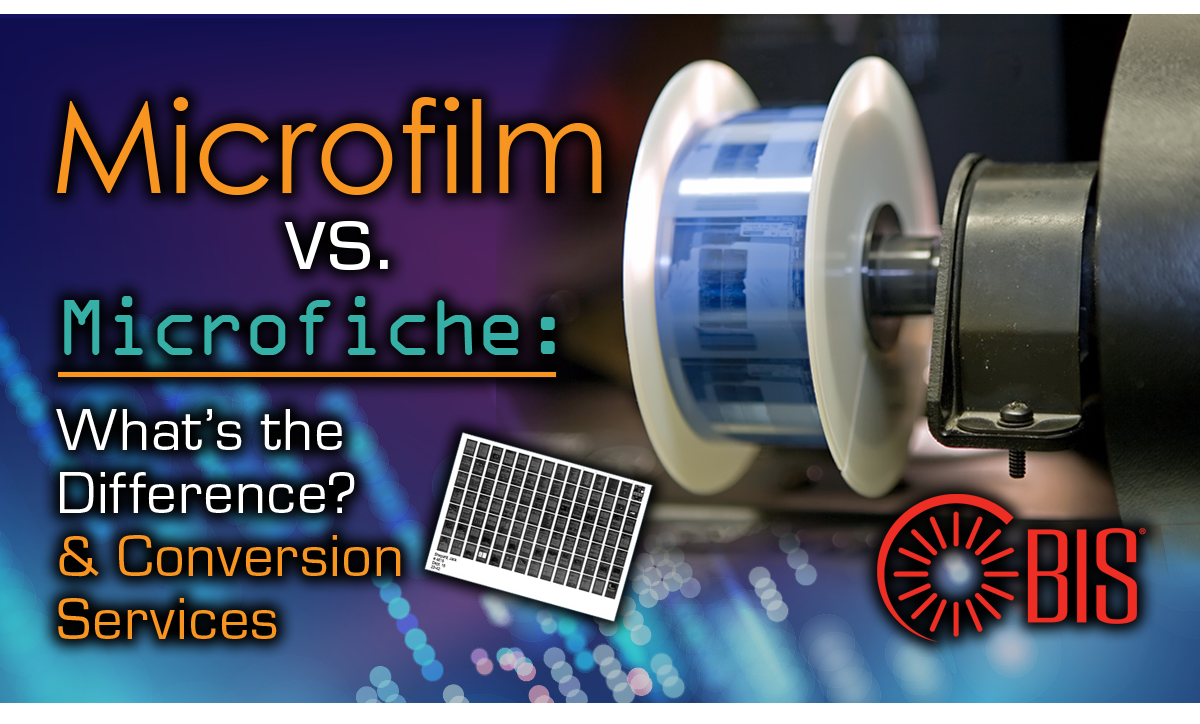The image appears to be an advertisement with a background gradient transitioning from dark purple to lighter purple and blue at the bottom. Blurry circular lights add a dynamic feel to the backdrop. Dominating the right side is a microfilm or microfiche machine, featuring two flat white cylinders with a transparent blue roll of tape between them, attached to a black component that appears to spin. Prominently displayed text reads "MICROFILM" in large yellow letters at the top, followed by "VS" in white, and "MICROFICHE" in turquoise. Below this, a yellow line separates the text "What's the difference in conversion services," with these words alternating between white and yellow colors. Additionally, there's an image resembling a white piece of paper with black squares, possibly small images, but the details are unclear. A logo is situated at the bottom right corner featuring red sun rays and the letters "BIS" in capitals, next to a design resembling a bullseye. The overall design suggests that this is an ad for a service comparing microfilm and microfiche, possibly a cover for a YouTube video or similar content.